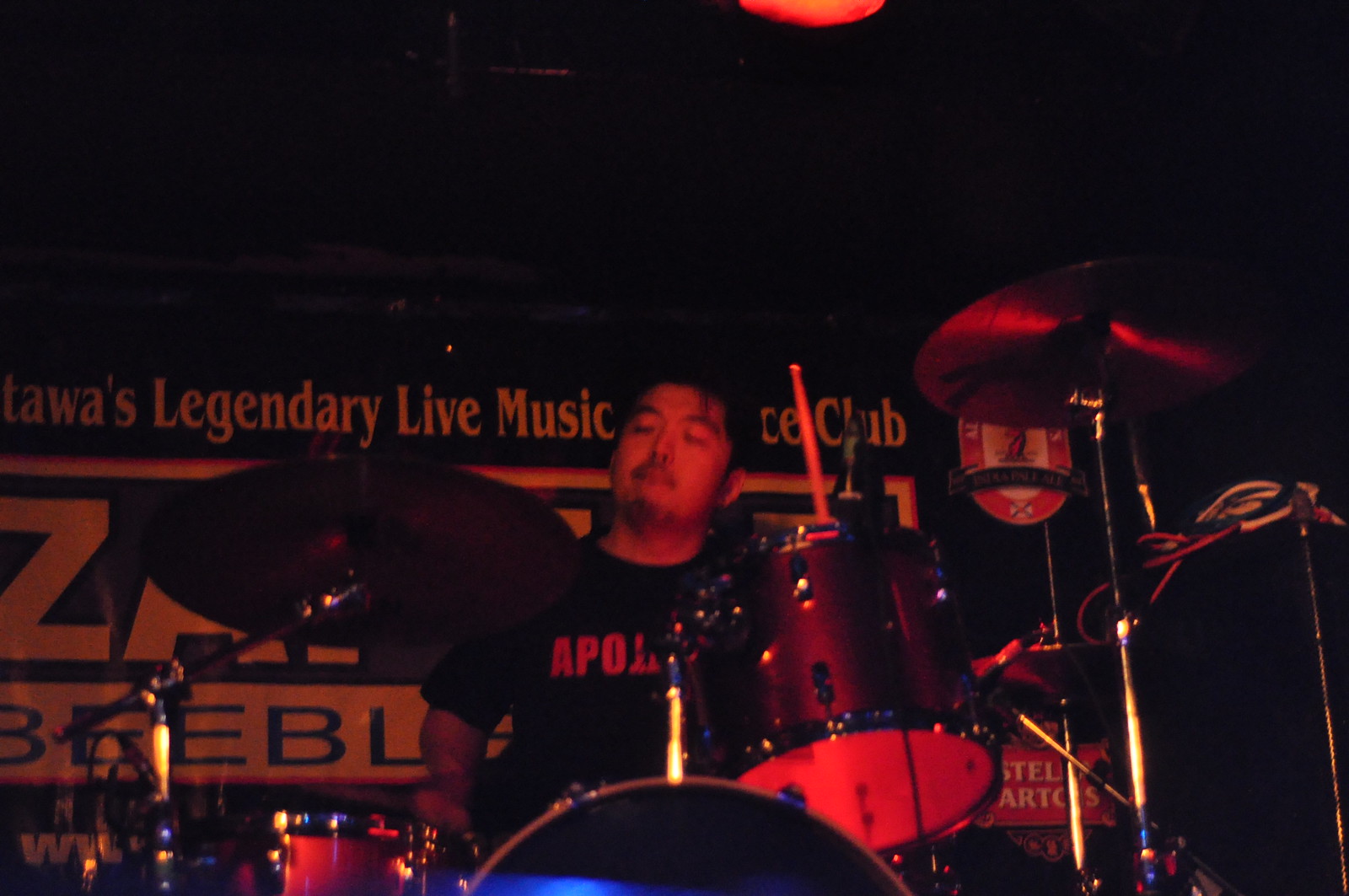In the dim lighting of a nightclub or music venue with a distinctive red glow, an Asian musician is captured deeply immersed in his drumming performance. The man, adorned with black hair, a solid mustache, and a separate beard, sits on a stage with his eyes closed, lost in the rhythm of the moment. He holds a drumstick aloft in his left hand, poised to strike. He wears a black t-shirt partially obscured by other objects, with only the letters "Apo" visible. The backdrop behind him, a black curtain with white text, partially reveals the phrase "legendary live music," while an advertisement for Stella Artois beer is subtly visible on a red background with white font. This scene, enveloped in darkness and red lighting, underscores the intensity and intimacy of the musical experience unfolding on stage.